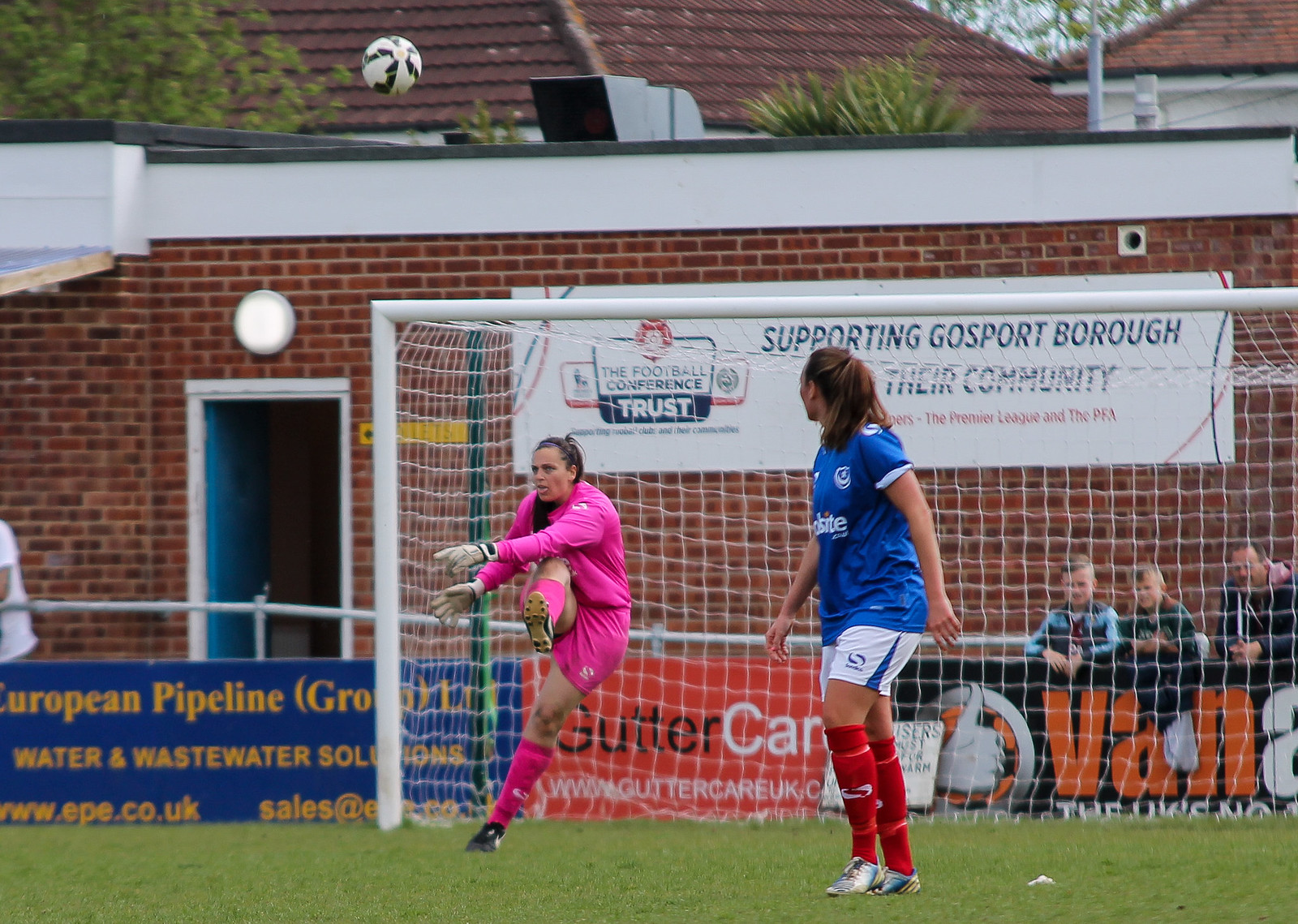The image captures an outdoor daytime soccer game on a green grass field, featuring two young women in action. At the foreground, a woman of Caucasian descent wearing a pink long-sleeved jersey, pink shorts, and pink knee-high socks is actively defending the white goal net; her right leg is raised, suggesting she has just kicked the white and black soccer ball, visible in the air above her. To her right, another woman, also of Caucasian descent, is watching the ball while facing slightly towards the camera. She is dressed in a short-sleeved blue jersey, white shorts, and red knee-high socks. Behind the net, there are three male spectators watching the game, seated in front of a low barrier adorned with advertising banners. In the background, a brick building and other structures with sloped roofs are visible. The banners include messages such as "Support GoSportBoro Community" and "European Pipeline."